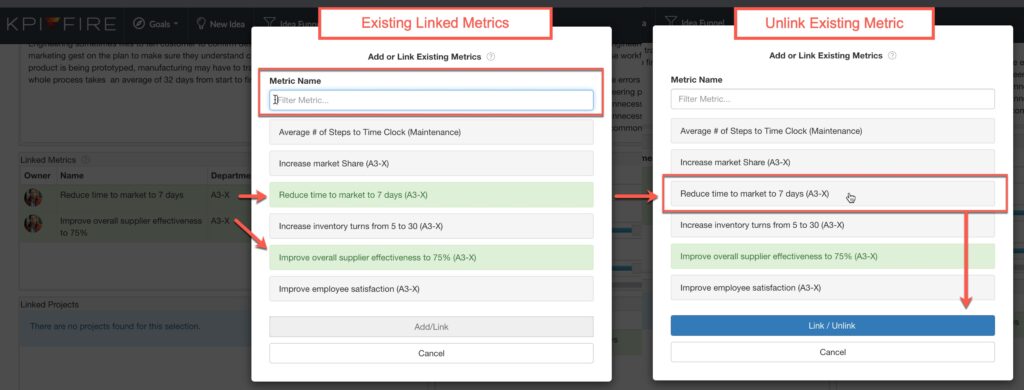The image depicts two pop-up windows superimposed over a grayed-out website background. Each pop-up window features a header with a red background. The right pop-up window is titled "Existing Linked Metrics" and displays a white interior with red text. On the left, the pop-up window reads "Add or Link Existing Metrics" and includes a detailed list of metrics, each enclosed with a red border, likely added through image editing.

Within the left pop-up window, the metrics listed are:
1. Average number of steps to time clock maintenance
2. Increase market share A3X
3. Reduce time to market to seven days A3X
4. Increase inventory from 5 to 30 A3X
5. Improve overall supplier effectiveness to 75%
6. Improve employee satisfaction

At the bottom of the left window, two buttons are visible: "Add Link" and "Cancel". Additionally, two red arrows are pointing to the options "Reduce time to market to seven days" and "Improve overall supplier effectiveness to 75%," both highlighted in green.

The right pop-up window appears to be the next sequential screen and is titled "Unlink Existing Metric". It emphasizes the "Reduce time to market to seven days" metric with another red border, and the "Unlink" button is highlighted in blue, accompanied by a red arrow pointing towards it.